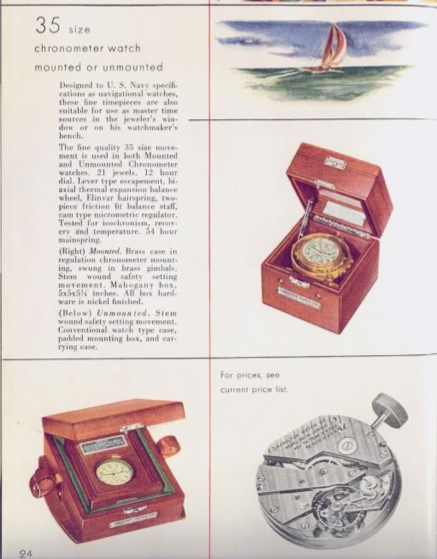This detailed illustration, likely from a mid-20th century book or magazine, depicts a "35 Size Chronometer Watch, Mounted or Unmounted" designed for U.S. Navy Pacific navigational purposes. The page number 24 appears at the bottom left, with the illustration including multiple visual elements. There's a watercolor painting of a sailboat against a green sea and dark blue sky at the top right. Below this, an open box reveals a chronometer watch with a gold-colored face, reinforcing its antique appearance, possibly dating back to the 1940s to 1960s. To the left of the box, another open box displays a similar watch face, further emphasizing the watch's historical design. Beneath these images, a detailed dissection of the chronometer watch, shaded in grayscale, reveals its intricate mechanical components. The overall presentation is supplemented by four paragraphs of text discussing the watch's design and quality, emphasizing its role in naval navigation.